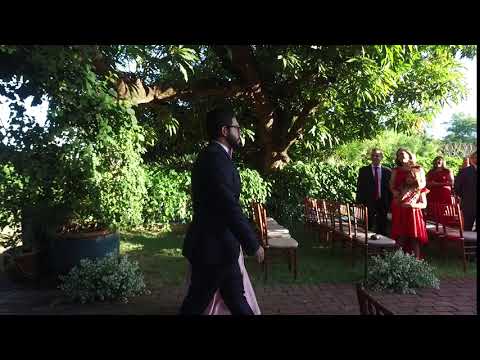This photograph captures a slightly blurry yet vibrant outdoor wedding scene set on a sunny day, with lush green trees enveloping the background and a significant large tree dominating the skyline. Centered in the frame, a man with dark hair, a black beard, and glasses is walking down a red brick aisle while wearing a black suit and white collared shirt. Though the bride is not in full view, the bottom of her dress can be seen beside him. The aisle is framed by rows of wooden chairs with white seats, occupied by elegantly dressed guests. Notably, some women in the crowd are wearing red dresses, holding flowers, and the men accompanying them are in dark suits with red ties. This picturesque setting underscores the joyous occasion, as the group solemnly observes the procession.